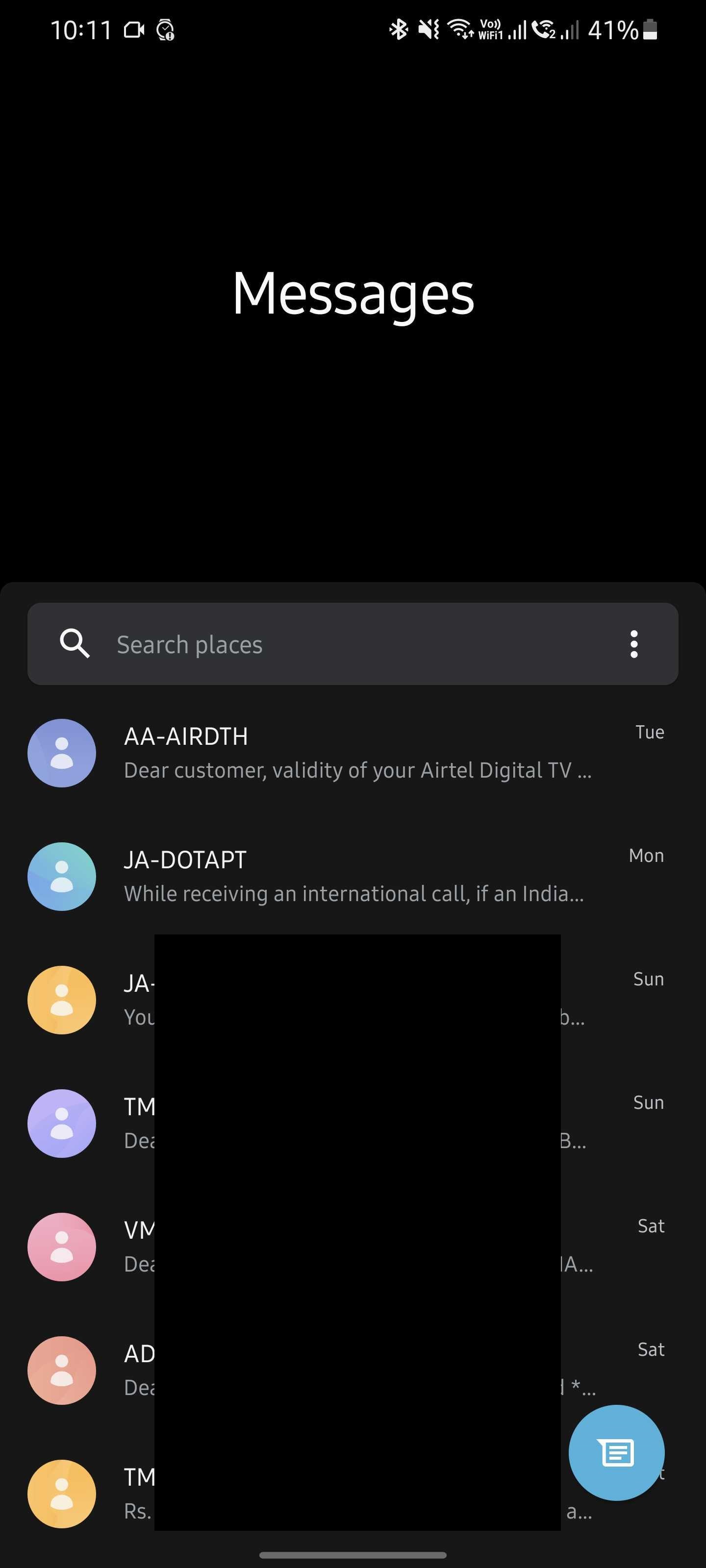A detailed view of a digital screen filled with various icons and notifications: prominently displayed are a video camera icon, an alarm clock, and Bluetooth connectivity. The screen indicates active Wi-Fi with 2 out of 4 bars and 41% battery remaining. Notifications and options include VoLTE Wi-Fi calling, message alerts, a search bar for places, and a menu represented by three dots. Text at the top mentions "AA, air, DTH," and a message to a customer regarding the validity of their Airtel digital TV service. Specific dates and abbreviations such as Tuesday, Sunday, Monday, Saturday, as well as names like "Tim" and "Vim," are also visible. There's a blue chat icon in the bottom right, while the middle section of the screen is obscured by a black square and a gray line runs horizontally at the bottom center. The brand "Airtel" appears multiple times throughout the display.